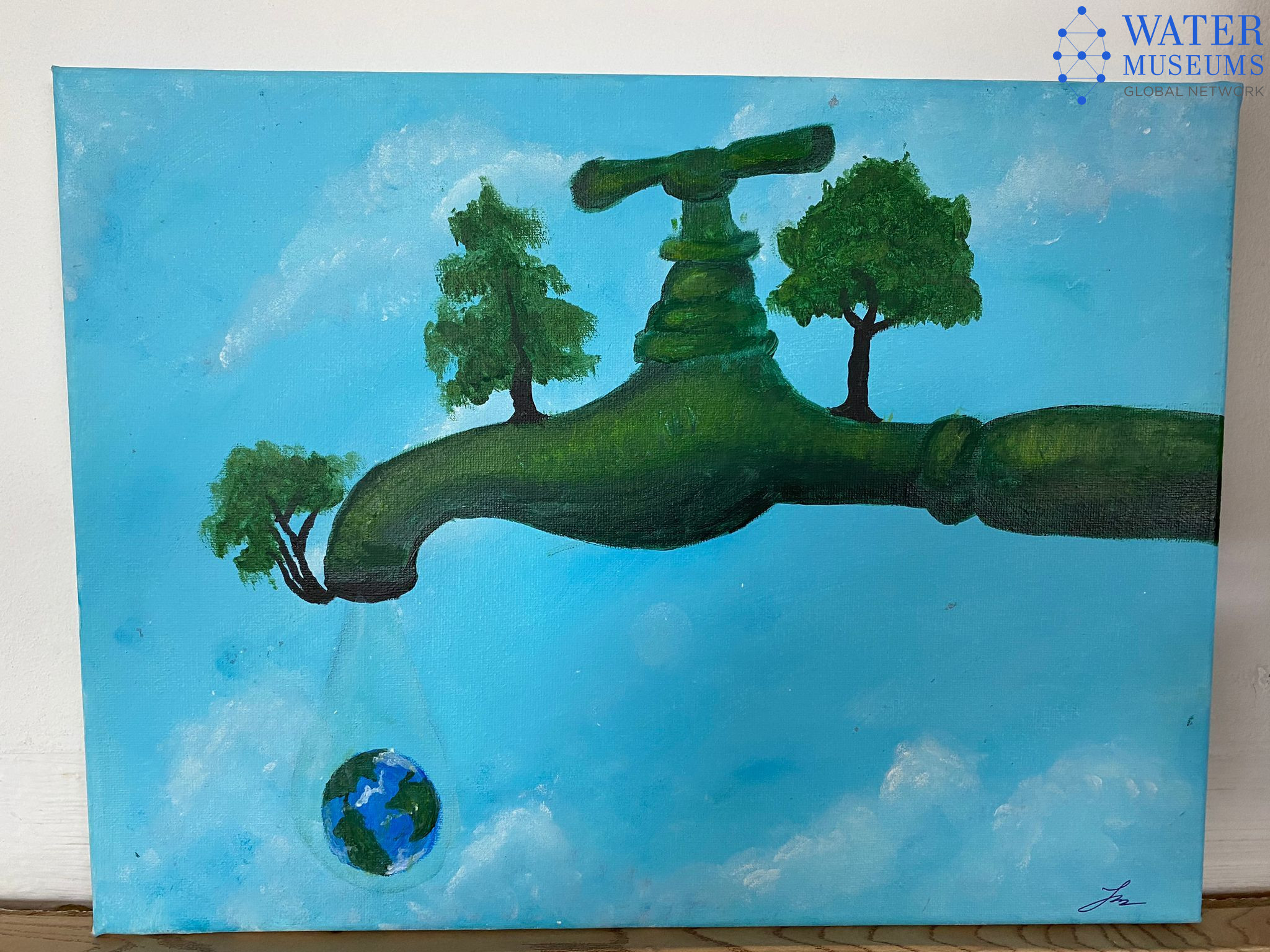The painting depicts a surreal image of a green faucet extending from the right side of the canvas, adorned with trees at various points. The green faucet, seemingly covered in moss or grass, stands against a backdrop of a bright blue sky dotted with white clouds. There are three distinct trees growing from it: a small leafy tree at the end where water would exit, an evergreen tree near the faucet's handle, and a larger shadowed tree behind the handle.

A significant feature is the droplet emerging from the faucet, encasing the Earth, which is depicted with blue and green hues representing oceans and continents. The painting is set against a light brown floor, leaning against a wall. In the bottom right-hand corner, the artist's signature is visible, and in the top right-hand corner, there is a watermark that reads "Water Museums Global Network," accompanied by a logo resembling an interconnected series of dots forming a teardrop shape.

Overall, the painting creatively combines elements of nature and human-made structures to deliver a message, possibly about environmental conservation and the interconnectedness of water and life on Earth.